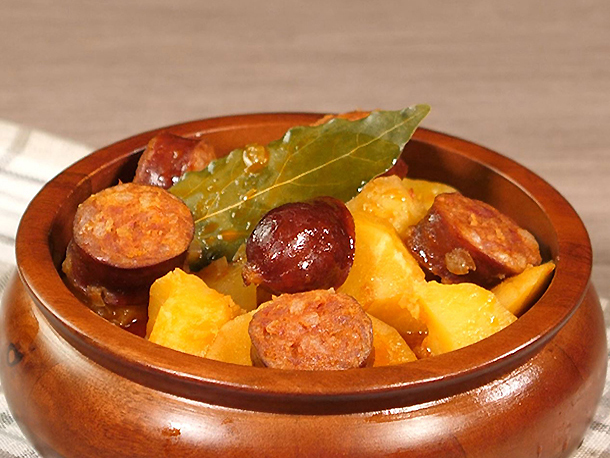This color photograph showcases a deliciously cooked meal presented in a round, shallow, brown terracotta bowl that gives the appearance of a small cauldron. The main ingredients visible include orange-brown, shiny, smoked kielbasa or sausage slices, mixed with chunky, cubed sweet potatoes or regular potatoes, and accompanied by pieces of what appears to be squash. A notable detail is a single bay leaf resting on top, garnished with a sauce, adding a touch of greenery to the ensemble. The food rests on a neatly patterned, light kitchen towel placed over a smooth, pale wooden table, with a slightly blurred grayish or tan surface in the background. The dish is devoid of utensils or hands, offering a clear, inviting view of the savory contents ready to be enjoyed.